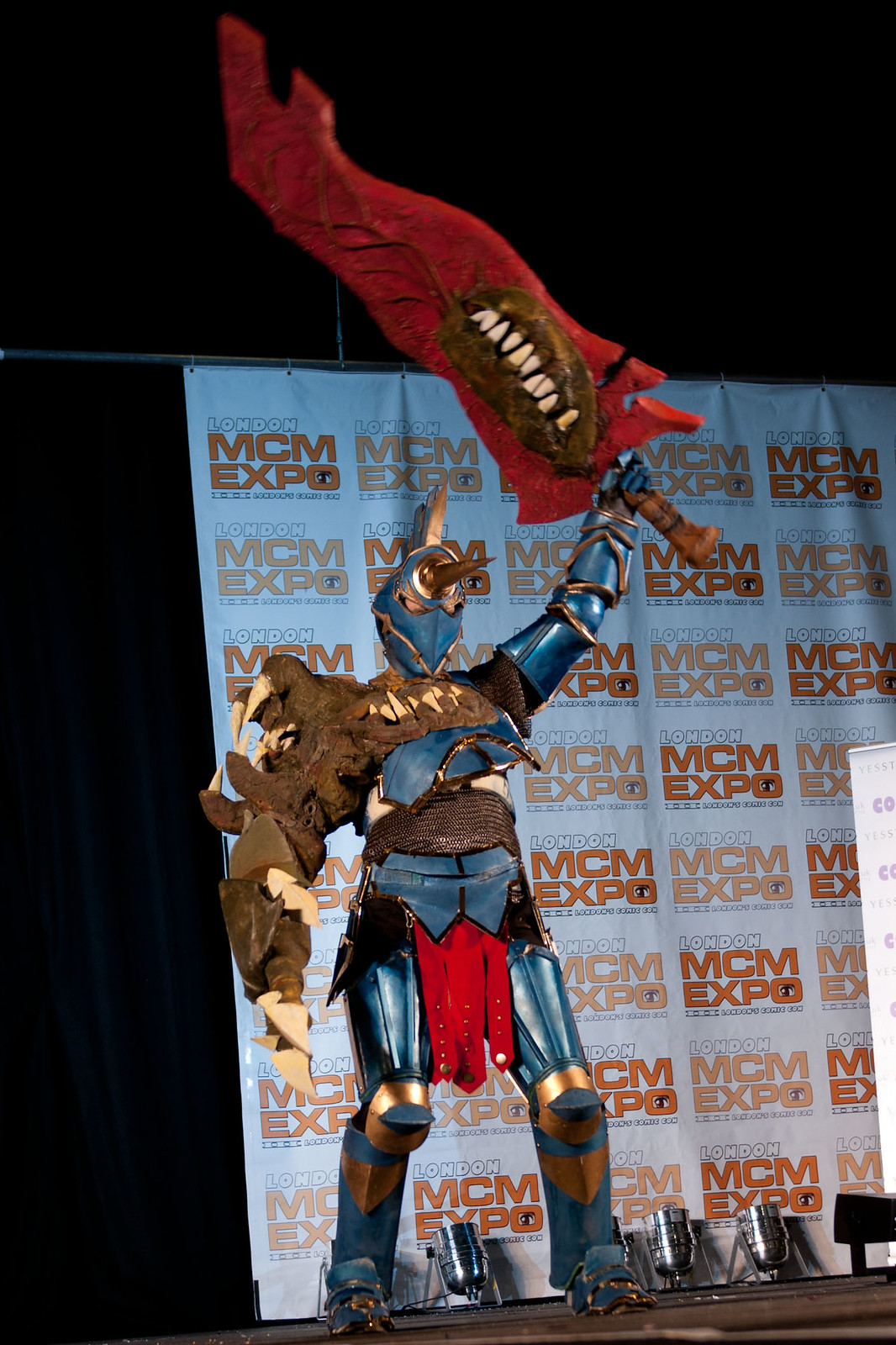The photograph captures a cosplayer dressed as a robotic warrior standing on stage at the MCM Expo in London. The backdrop prominently features the event's name "MCM Expo" repeatedly in alternating red and yellow fonts, highlighted by multiple spotlights. The cosplayer's intricate costume is primarily blue armor, accented with gold details around the elbows, wrists, knees, shins, and jaw area. He wears a helmet adorned with a prominent rhinoceros-like horn and spikes on top. His right arm is designed to resemble the limb of a dinosaur or creature, complete with claws from the shoulder to the hand. Draped across his middle is a red loincloth with a hint of chainmail, while his left arm wields a dramatic, large red sword with a mouth-like design near the hilt. The armored suit, evocative of an upgraded knight from a video game, seamlessly blends human and creature elements, making for a striking and memorable cosplay display.